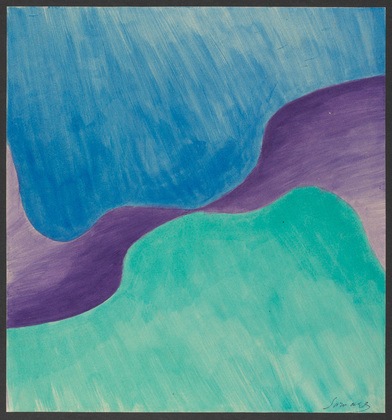The image depicts a simple, abstract watercolor painting characterized by three main hues: blue, purple, and lime green. The canvas is divided into three distinct sections with the top portion painted in various shades of blue, resembling a sky with visible white streaks where the paint isn't fully filled in. Below the blue is a flowing, ribbon-like wave of purple that stretches across the width of the image, starting wide, tapering to a thin line in the middle, and then widening again. This purple wave demonstrates a gradient of shades, transitioning from light lilac and lavender to dark plum. The bottom section of the painting showcases a light lime green color, irregularly filled in with noticeable white patches, giving it a scribbled, unrefined look. In the lower right corner, there's an etched signature by the artist, somewhat illegible but identifiable by an 'S.' The overall appearance suggests an abstract scene, possibly depicting a blend of natural elements like sky, land, and water, unified by a flowing purple ribbon. The brush strokes appear amateurish, reinforcing the painting's simplistic yet dynamic nature.